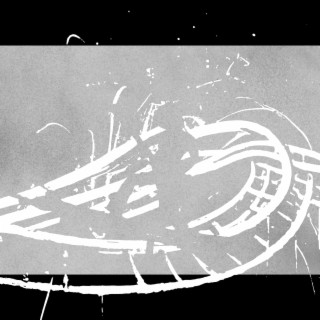The image is a still from a video, presenting an abstract, monochromatic scene. It features a gray background, flanked by black letterbox bands at the top and bottom. Dominating the center are intricate white lines forming a complex, spiraling pattern reminiscent of train tracks or a circular staircase. Implied within this swirling design is the faint silhouette of a person playing a guitar, their pose suggesting a concert performance with one leg elevated higher than the other. Scattered across the image are white specks, adding to the dynamic feel, possibly evoking the impression of fireworks. The overall composition has a 3D appearance, with an oval shape intersected by vertical lines, creating a layered, multidimensional effect.